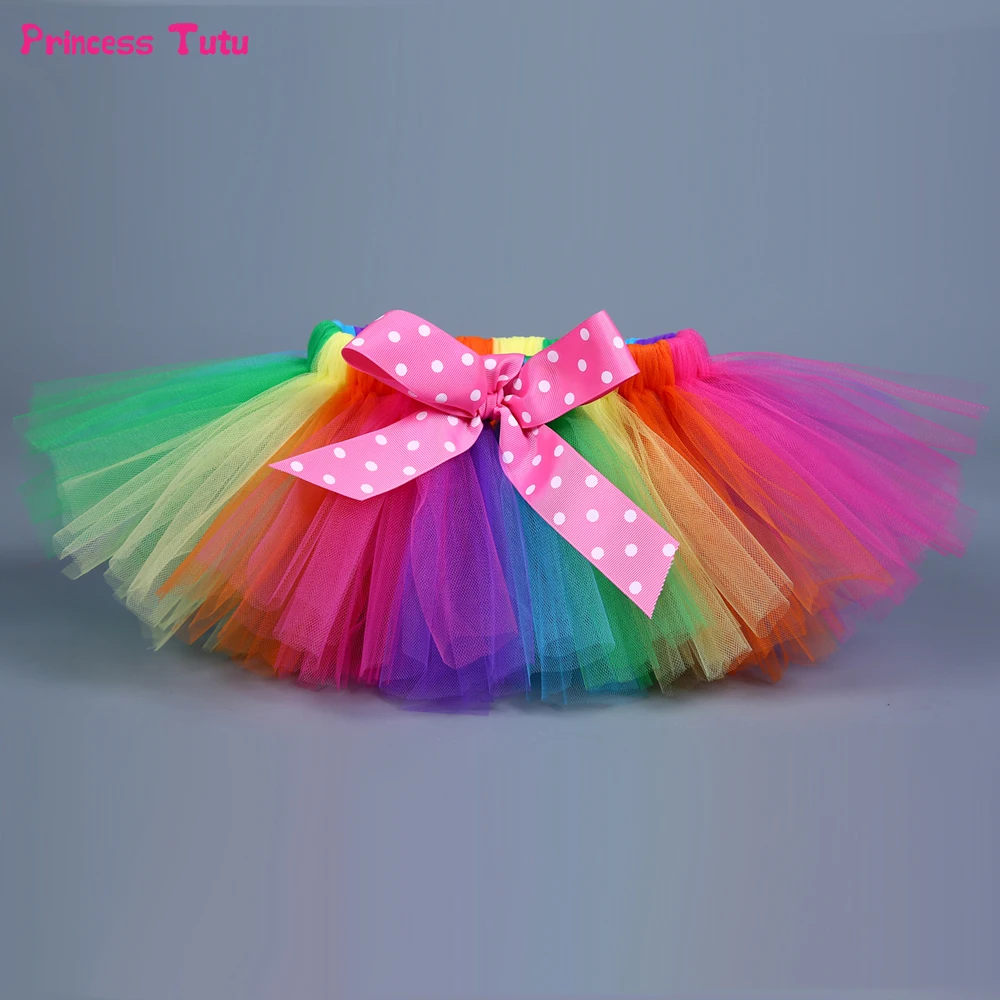The square image, measuring approximately six by six inches, features a dark gray background. In the upper left-hand corner, bold pink sans-serif text reads "Princess Tutu," casting a subtle shadow on the backdrop. Centrally placed is a fluffy, horizontally-aligned, multicolored tutu. A large, hand-tied, light pink bow with white polka dots sits prominently at the front of the tutu. The tutu is layered with rainbow-colored lace arranged sequentially from left to right: green, yellow, orange, purple, blue, a different shade of blue, then repeating with green, yellow, orange, pink. The waist area at the back of the tutu continues this color pattern, hinting at an orange, yellow, and green combo even though the lace from this side isn't fully visible. Shadows under the tutu suggest a light source from the upper area, with darker shading towards the lower left and right sides. The design and text, combined with the vibrant colors, evoke a whimsical and playful feel appropriate for a little girl's ballet outfit.